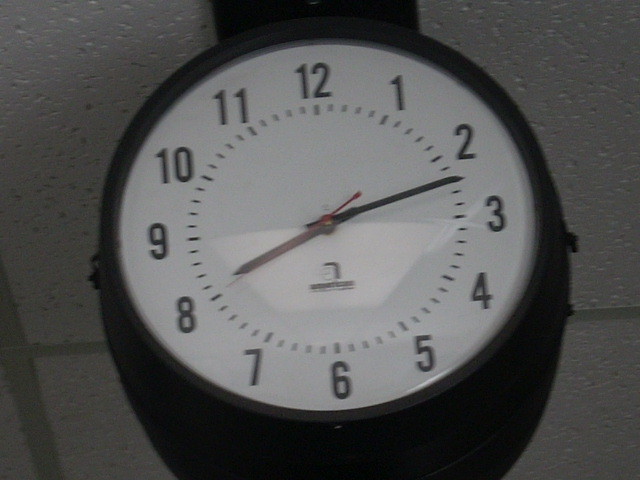The photograph features an industrial-style ceiling clock mounted on a ceiling made of white acoustic paneling. The image is dimly lit, suggesting that the room's lighting is not fully illuminated. The clock itself is robust and black, contrasting starkly against the white background. Its face is white with standard Arabic numerals from 1 to 12 clearly marked in their usual positions. The clock has black hour and minute hands, complemented by a red second hand, which adds a pop of color. The time displayed on the clock is 8:12.